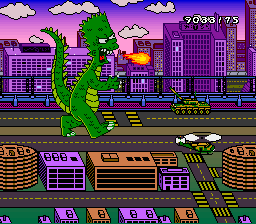This image appears to be a still from a vintage 8-bit style video game with a slightly pixelated look. The scene is set against a vibrant backdrop featuring a pink and blue sky dotted with white clouds. The cityscape includes boxy purple and orange buildings that line the horizon. A large green Godzilla-like monster dominates the scene, walking to the right on a four-lane road. This creature, with a head resembling Bart Simpson, is dark green with a lighter green underside, sharp white claws, and white tail spikes. It is depicted breathing a bolt of fire or fire torpedo from its open mouth, which displays sharp teeth and a red tongue. Green camouflage helicopters and tanks point toward the monster, adding to the chaotic atmosphere. A numerical code, 9033-75, is displayed in white font in the top right corner. The overall color scheme of the image merges purplish, brown, and pink tones with some green accents in the background.